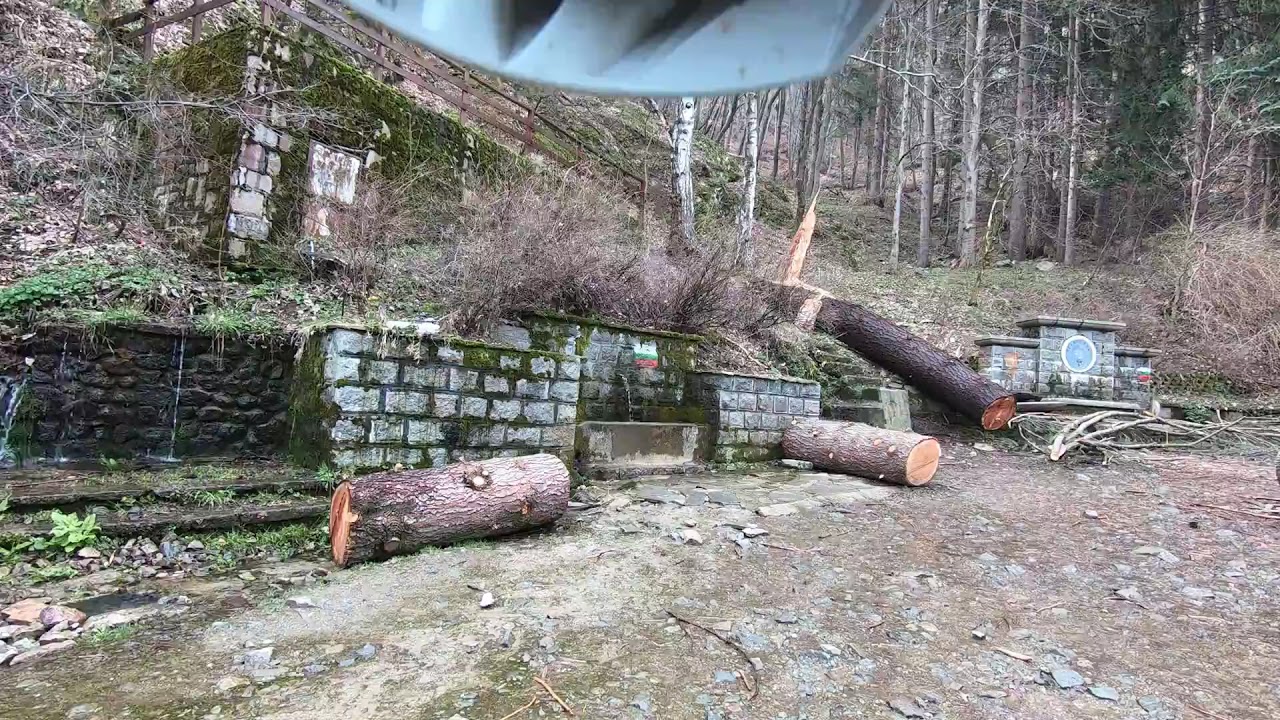The image captures a serene, outdoors nature area, devoid of any human presence. The foreground features a dirt-covered ground, scattered with grey rocks, trampled leaves, and stray twigs. Prominently lying on the ground are three neatly cut logs, one larger than the others, showcasing their light coffee brown interiors and darker exteriors. These logs are positioned near a series of moss-covered, old stone masonry walls that jut out at various angles. Towards the left side of the image, some of these walls support a wooden handrail composed of three boards, which extends up a grassy bank and further connects to stone steps that appear to lead upwards. In the far background, a mix of deciduous and evergreen trees, most of which are leafless, stand tall against a backdrop of timber, suggesting past logging activity. Additionally, a sloping mountain adds to the rugged charm of the scene. At the very top of the image, a sliver of metal or plastic, white in color, intrudes into the frame, adding a modern yet cryptic element to this otherwise rustic landscape.